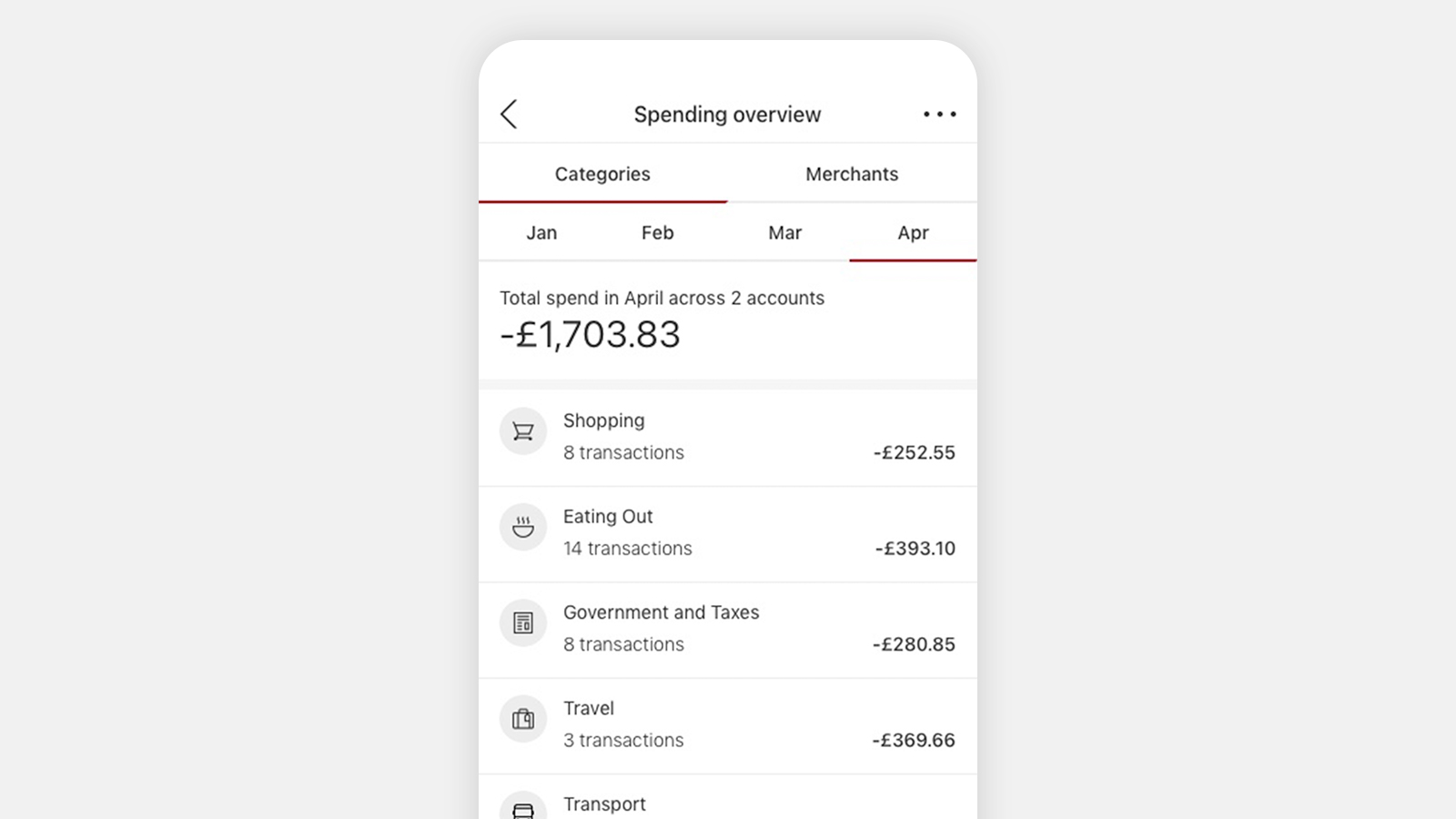**Detailed Caption:**

The image showcases a screenshot of a spending overview displayed on a smartphone. The interface features a clean design with black text on a white background. At the top of the screen, "Spending Overview" is prominently displayed, flanked by a back button on the left and a context menu icon on the right. Below this heading, there are two tabs labeled "Categories" and "Merchants." The "Categories" tab is underlined in red, indicating it is currently selected.

Further down, a navigation menu lists the months of January, February, March, and April. April is underlined in red, specifying it is the active month. The total spend for April across two accounts is reported as -£1,703.83.

The breakdown of expenditures in April is as follows:
- **Shopping:** 8 transactions totaling -£256.25.
- **Eating Out:** 14 transactions totaling £393.10.
- **Government and Taxes:** 8 transactions totaling -£280.85.
- **Travel:** 3 transactions totaling -£369.66.

There is an additional category for "Transport" that seems to be cut off at the bottom of the screen. This financial tracking application highlights the user's spending patterns, revealing significant expenses, particularly in dining out, which amount to a notable sum for a single month.